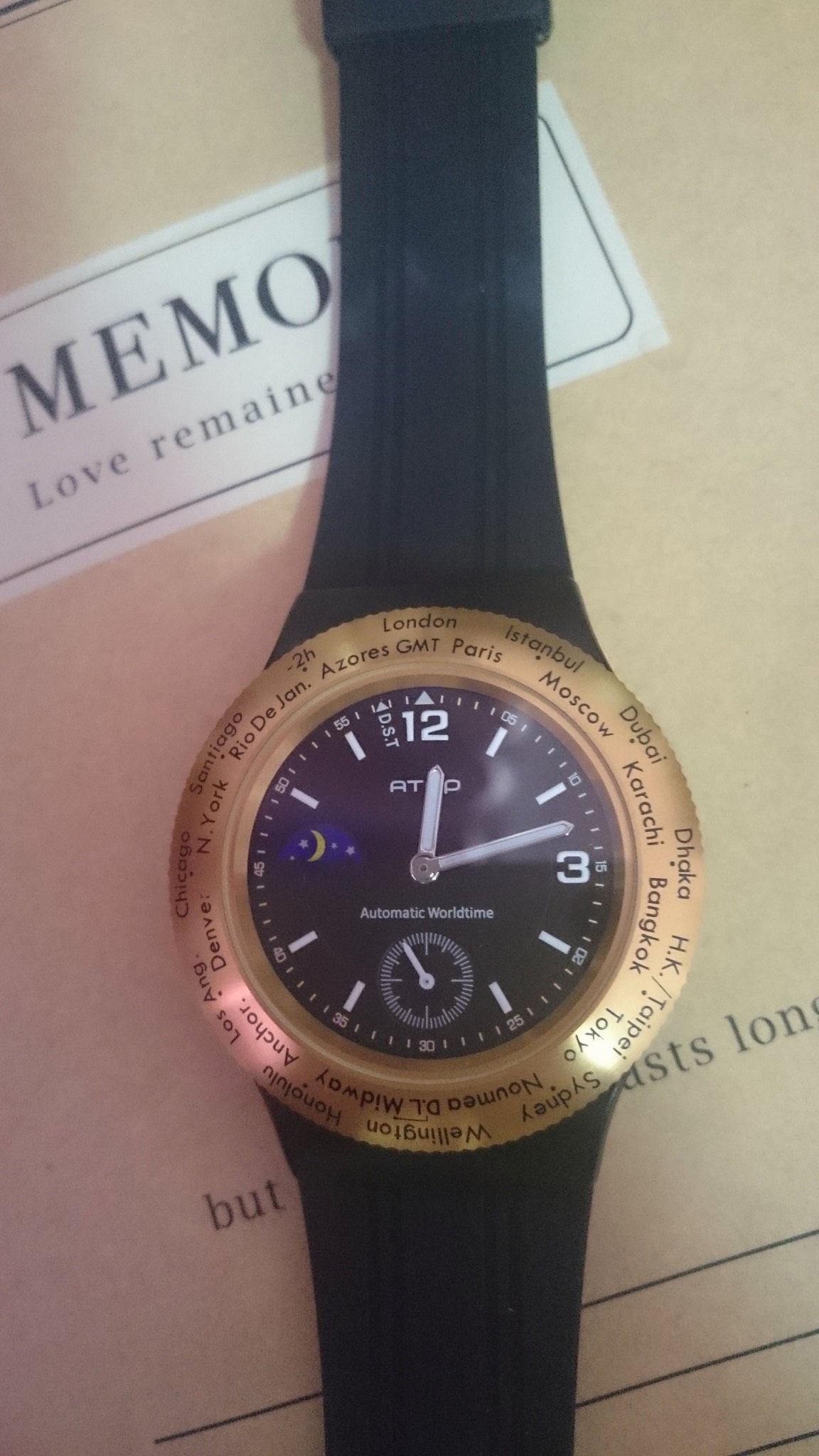A detailed image of a wristwatch resting atop what appears to be a tan-colored piece of paper or perhaps a folder labeled "MEMO." The watch's navy blue band partially obscures the writing, which also includes the phrase "love remains" in black print within a white text box. At the document’s bottom, the words "BUT" and "LONG" appear in black print, separated by an array of straight lines. The watch dial is adorned with a gold bezel featuring the names of famous cities such as London, Paris, Moscow, Dubai, Bangkok, Tokyo, Wellington, Sydney, Honolulu, Los Angeles, Denver, Chicago, Santiago, New York, and Rio de Janeiro. The watch face is marked with hash marks for the hours, but only the 12 and 3 positions are adorned with numerals.